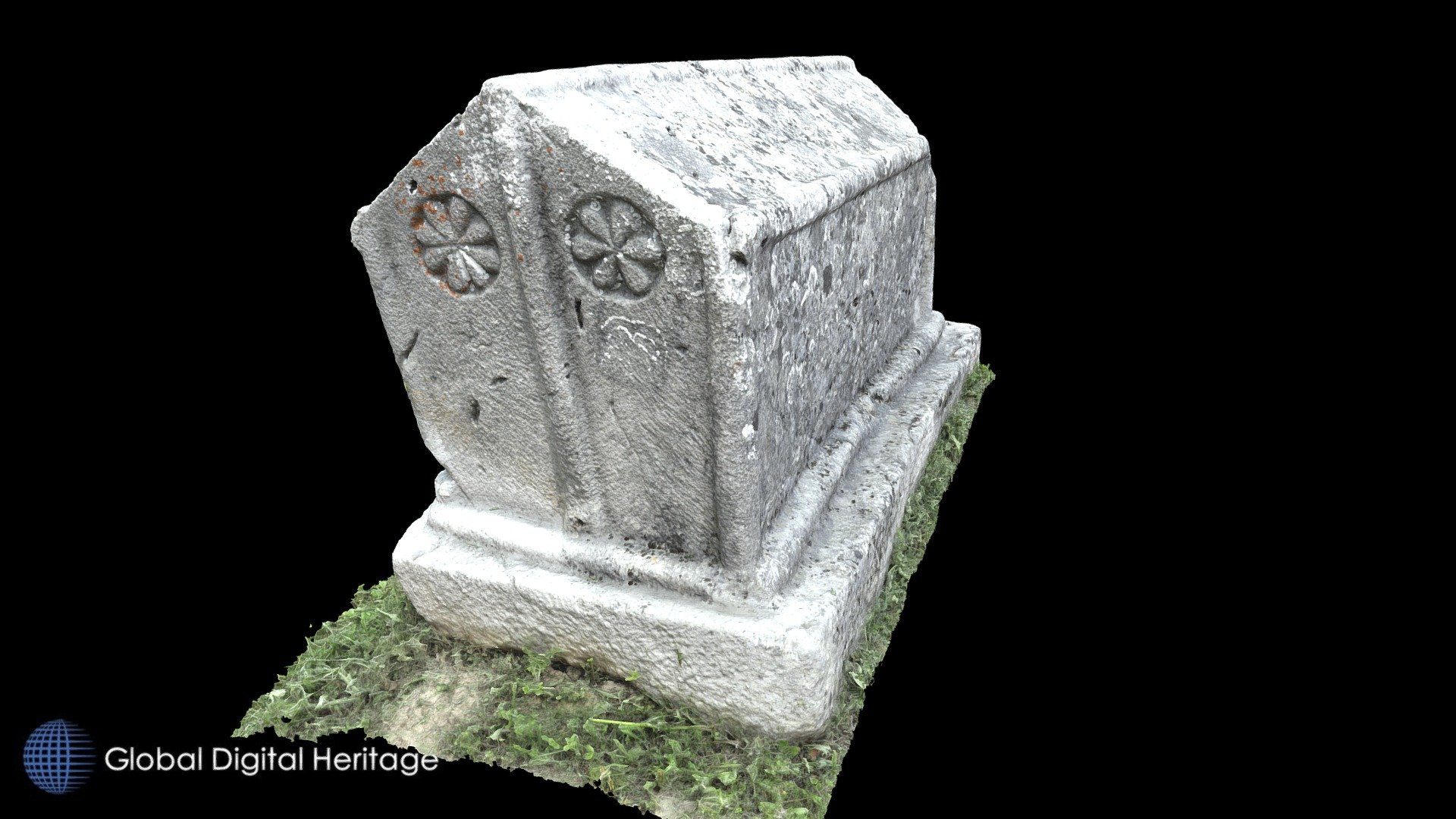This image showcases an intricately designed tomb or grave, sculpted from gray stone. It features a long, rectangular base that resembles white concrete, providing a sturdy foundation. Atop this base sits a structure shaped like a small house, characterized by a smooth wall on its right side and a slanted roof. The front facade of this house-like structure is pointed at the top, with a prominent vertical line running centrally from top to bottom. Flanking this line are two ornate flower medallions, one on each side, adding decorative detail to the solemn monument. The tomb rests on a bed of grass, contrasting sharply with the pitch-black background that envelops the scene. The lower left corner of the image bears the inscription "Global Digital Heritage."